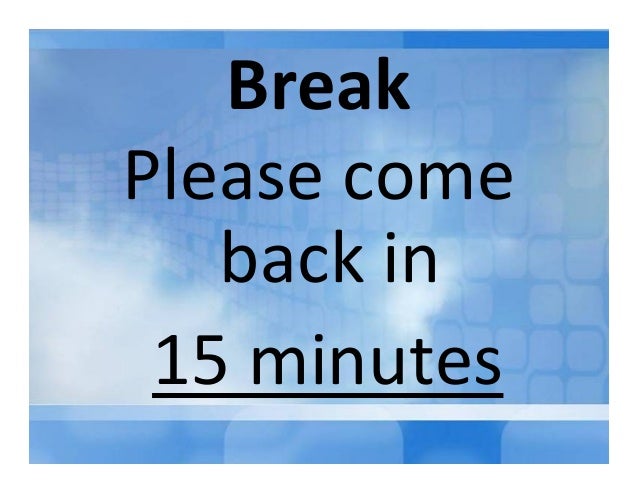The image is a color infographic in landscape orientation, featuring a mostly blue background adorned with a checkered tile pattern of varying blue shades, giving it a graphic texture. A light white tint overlays the midsection, with a white clouded image on the left side, creating a subtle gradient effect. At the top center of the image, "BREAK" is prominently displayed in bold, black text. Directly below, in a medium-weight black font, the text reads, "Please come back in 15 minutes," with "15 minutes" underlined for emphasis. The entire composition is framed by a thick white border, and a distinctive band at the bottom transitions from white on the right to blue on the left, enhancing the infographic design's visual appeal.